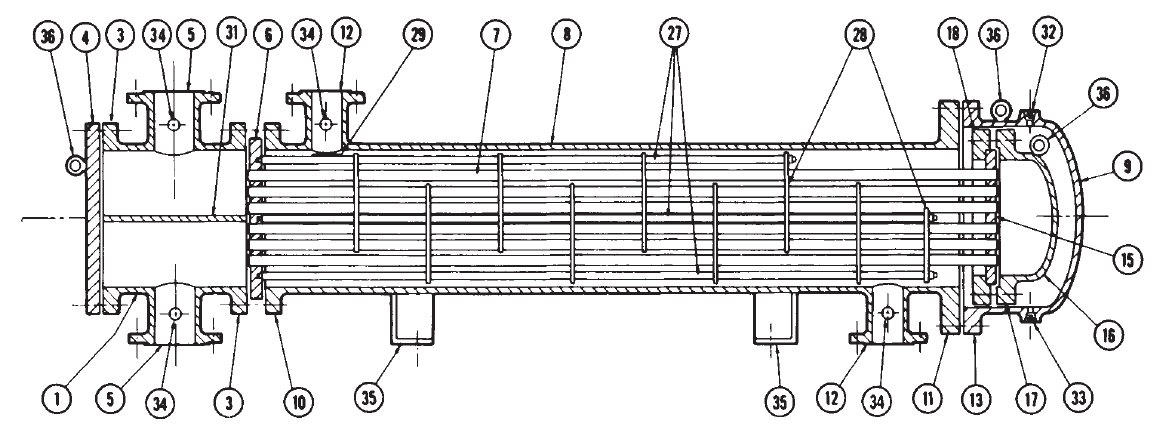This is a black and white rendered image, possibly illustrating a diagram of a construction plan, a map, or instruction manual for assembling machinery. The image is a long, slender rectangle oriented in a landscape format, featuring a primary rectangular object that has various protrusions and alcoves, resembling a cathedral with smaller adjacent sections. The right side of the main object is notably rounded. The diagram is detailed and numerically labeled, with numbers ranging from 1 up to around 36, each enclosed in a circle and connected to specific spots on the diagram by lines. The central part includes several connecting tubes, some running horizontally between the two sides and others vertically along the structure. There is no key provided to explain the labeled numbers, leaving their specific meanings unclear.